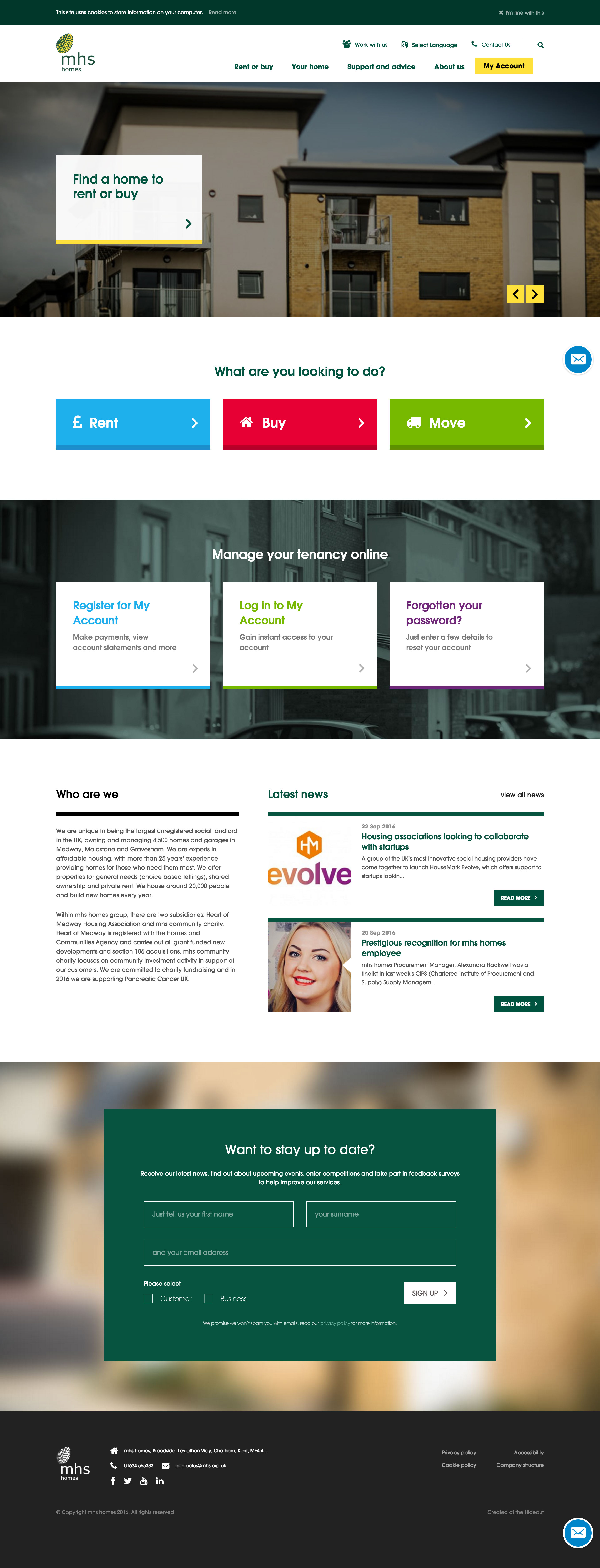The image features a house apartment building set against a white background. In the foreground, there are three prominent colored rectangles: the first one is blue and labeled "Rent," the second is red labeled "Buy," and the third is green labeled "Move." Additionally, within the image, there is a section titled "Who Are We" accompanied by a picture of a smiling woman. She has red lipstick and her teeth are visible. Adjacent to her image, there is a green rectangle titled "Evolve," which contains related information. Below this, there is another green rectangle featuring checkboxes paired with corresponding information. There is also a white rectangle with a small, green text—possibly "Register," although it is not entirely clear due to its size. The bottom portion of the image has a black area.